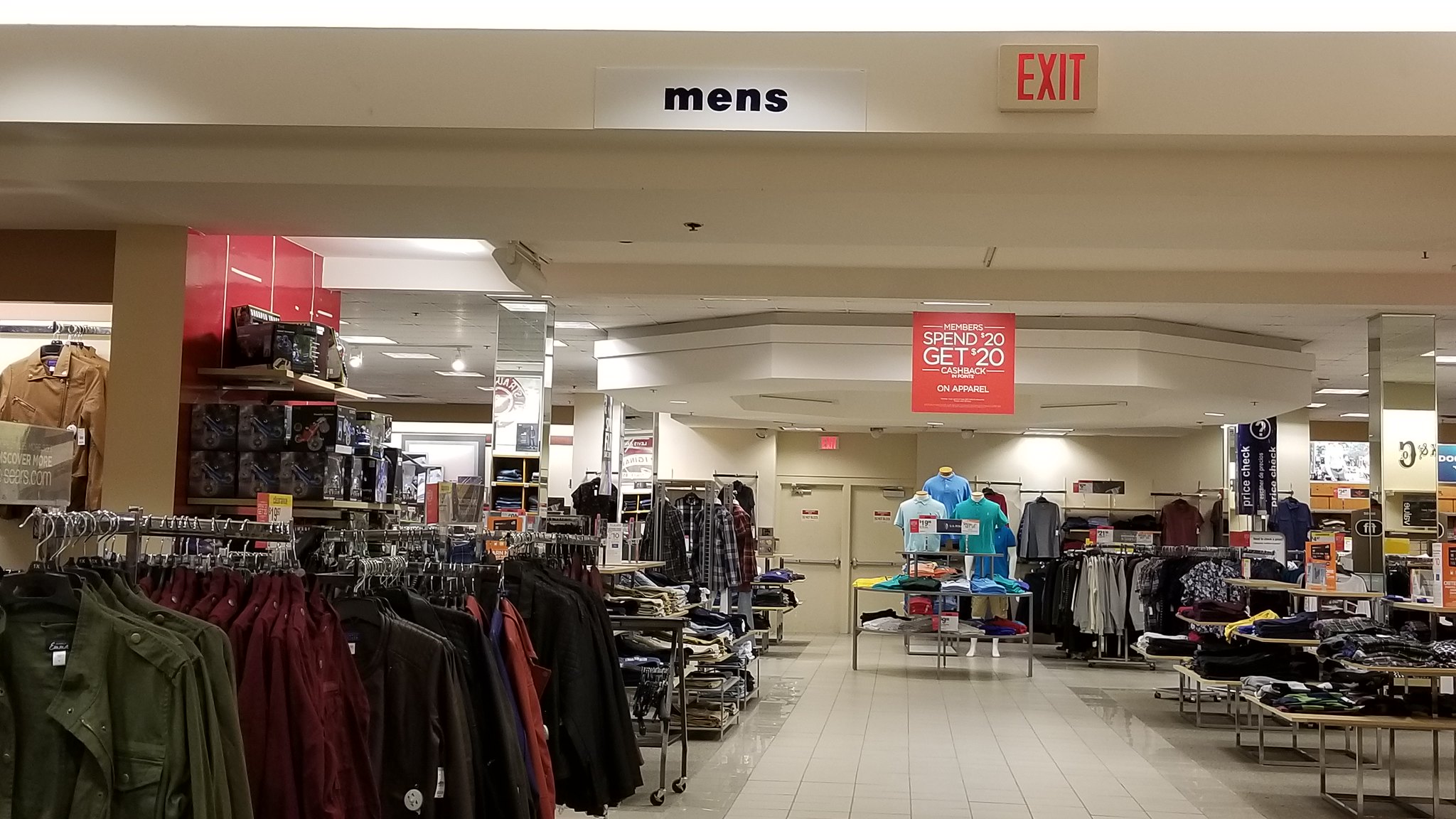This image captures the interior of the men's department in a bustling department store. Directly ahead, we see a spacious open aisle flanked by organized racks of men's clothing and accessories on both sides. At the top of the image, an archway features a prominent red exit sign next to the word "Men's" in bold lettering.

Further down the aisle, a red promotional sign hangs, announcing an offer: "Spend $20, Get $20." This enticing deal draws the eye towards the central focal point of the department: a table display featuring several torso mannequins adorned in various shades of blue polo shirts. Surrounding the mannequins, shelves are neatly stocked with folded polo shirts in an array of colors, creating a vibrant and inviting display.

To the right of the aisle, a rack is filled with an assortment of hanging shirts and jackets. Beyond this, additional shelves hold more men's apparel, ensuring a wide selection for shoppers. On the left side of the aisle, there are numerous shelves and racks, each meticulously arranged with a diverse range of men's clothing, further enhancing the department's well-organized and appealing atmosphere.